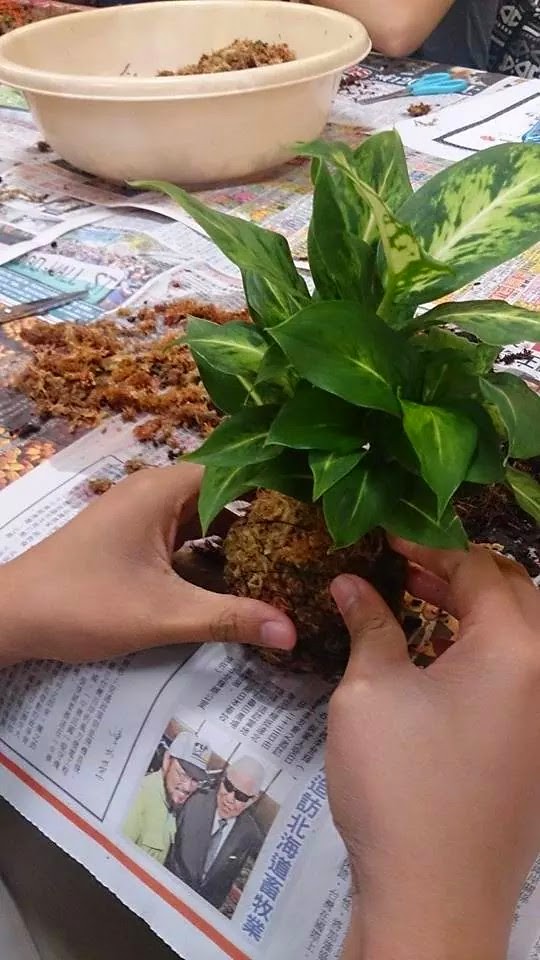The image captures the meticulous hands of a young person, engrossed in transplanting a small plant with vibrant green, teardrop-shaped leaves. The scene unfolds on a table draped with what appears to be Korean newspaper, hinting at an international backdrop. Prominently in the foreground, the young hands work carefully, gripping the dirt and roots surrounding the plant. A white or tan bowl filled with dirt or mulch is placed on the newspaper-covered table, alongside a pair of scissors, possibly used for trimming the roots or soil, evidenced by the small pile of dirt or plant trimmings nearby. In the background, only an elbow of another person is visible, indicating that at least two individuals are involved in this gardening activity, likely preparing to transfer plants between pots or basins. The rich details and the concentrated effort depicted in the hands highlight a moment of thoughtful and collaborative gardening.